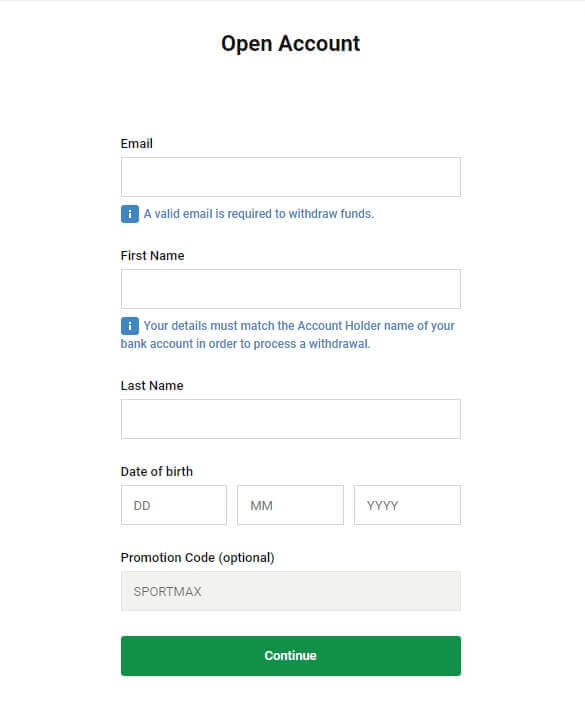Screenshot of a tablet screen displaying an online account opening form. At the top center, there is a header in bold black text that reads, "Open Account." Below the header is a form consisting of several fields. The first field is labeled "Email" in bold black text, with a white input box beneath it. A note under the input box specifies, "A valid email is required to withdraw funds." 

The next field is labeled "First Name" in bold black text, with a corresponding white input box below it. An instruction beneath this box states, "Your details must match the account holder name of your bank account in order to process a withdrawal."

Following this is the "Last Name" field, also in bold black text, with its white input box placed below. 

Finally, there is the "Date of Birth" section, denoted in bold black text, followed by three white input boxes labeled "DD," "MM," and "YYYY," for day, month, and year respectively.